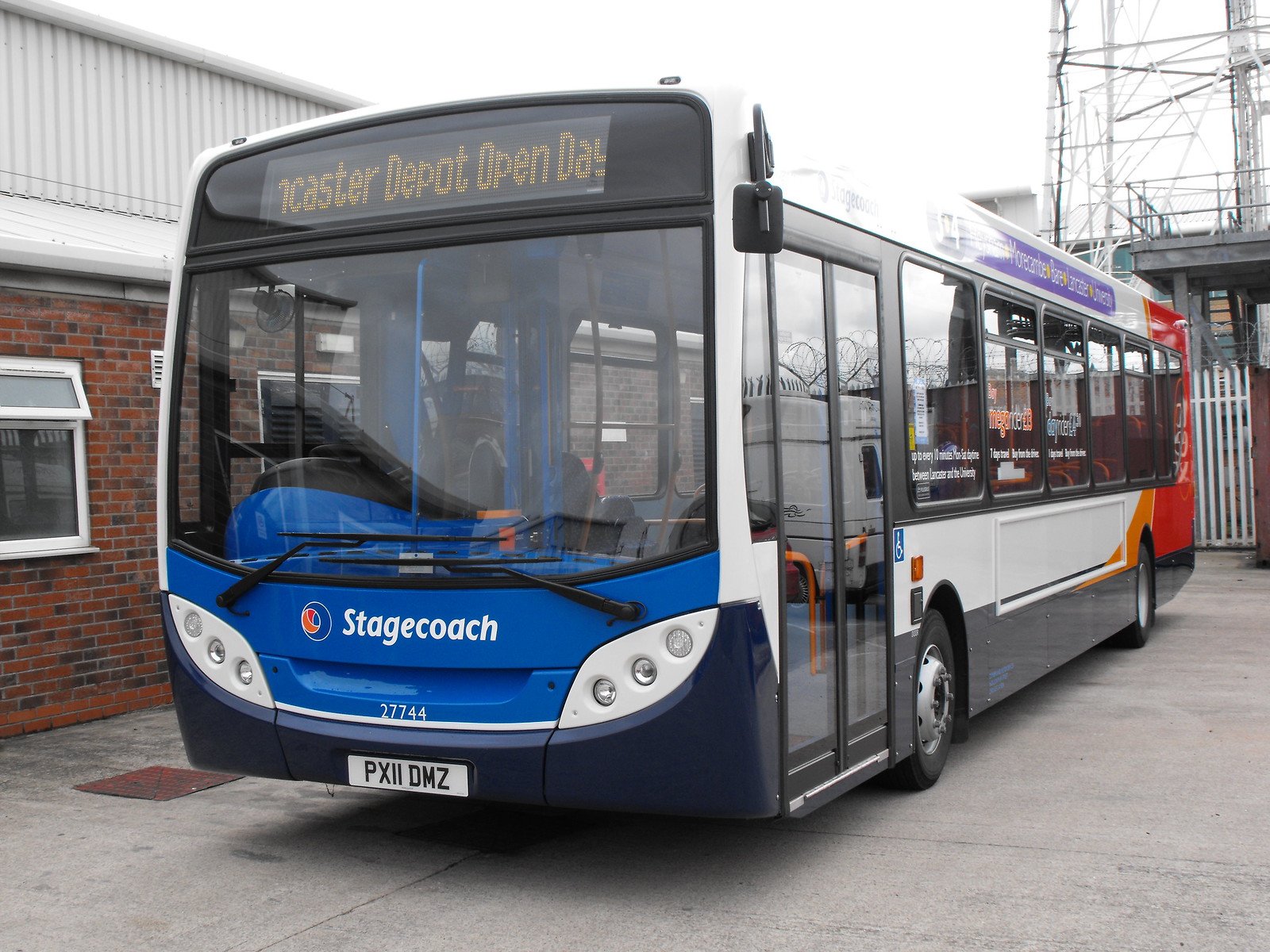This photograph captures a blue Stagecoach bus, prominently featuring various shades of blue with white stripes along its side. Parked at one of its stops, the bus displays a banner at the top that reads "Doncaster Depot Opening Day." The digital sign on the front, though partially cut off in this still image, matches the Doncaster location noted. Below the banner, two large windshields with wipers are visible, and the bus brand "Stagecoach" can be seen clearly. The license plate reads PX11 DMZ, indicating it is not from California, despite initial confusion with the Lancaster name. Additional writing adorns the side windows, and an advertisement runs vertically down the left side of the bus. The bus number is 27744, adding to the detailed identification of the vehicle.